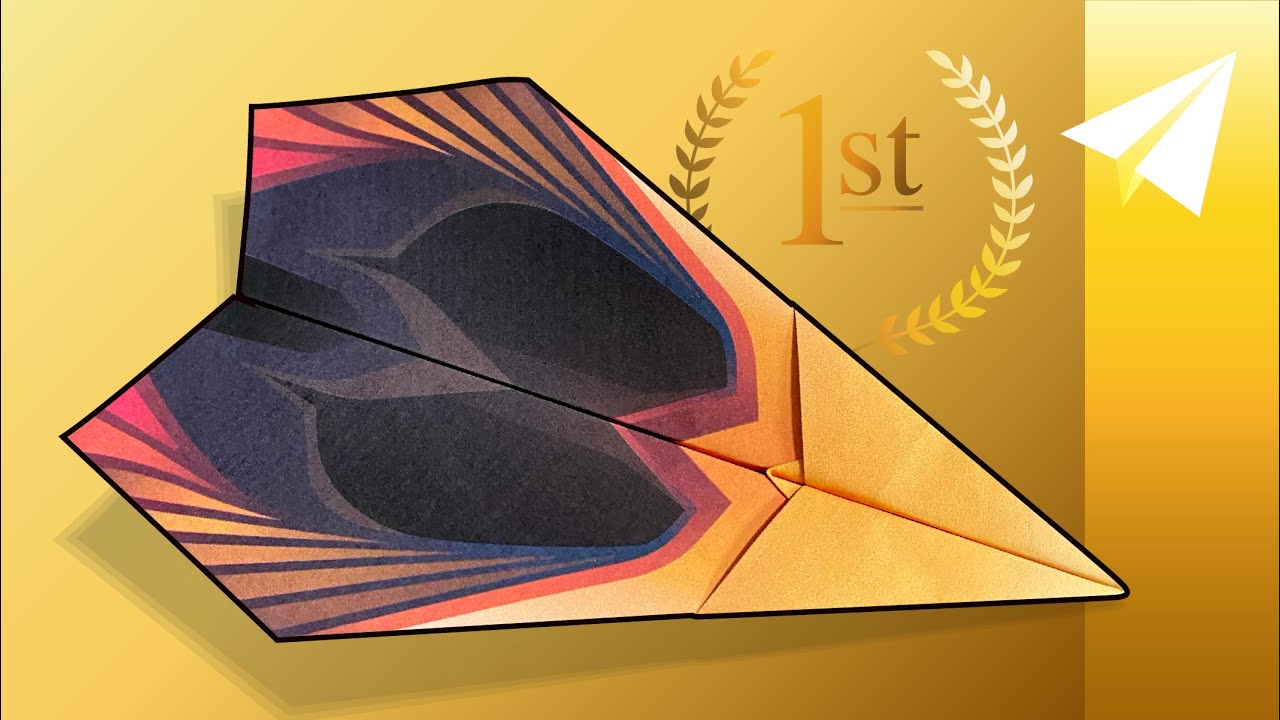This digital artwork features a predominantly gold background with an ombre effect, transitioning from a lighter shade on the left to a deeper hue on the right and bottom. At the center is a stylized origami paper airplane, outlined in black with a detailed shadow that gives it a three-dimensional appearance. The wings of the airplane are intricately designed with patterns resembling peacock feathers, incorporating dark blue, gray, red, orange, and yellow colors. Above and slightly to the right of this central airplane, the number "1ST" is emblazoned within a gold laurel wreath, indicating an award. Additionally, in the top right corner of the image, a smaller white paper airplane points upwards, reinforcing the motif. The overall composition melds drawing and digital elements, creating a uniquely vibrant and dynamic visual.